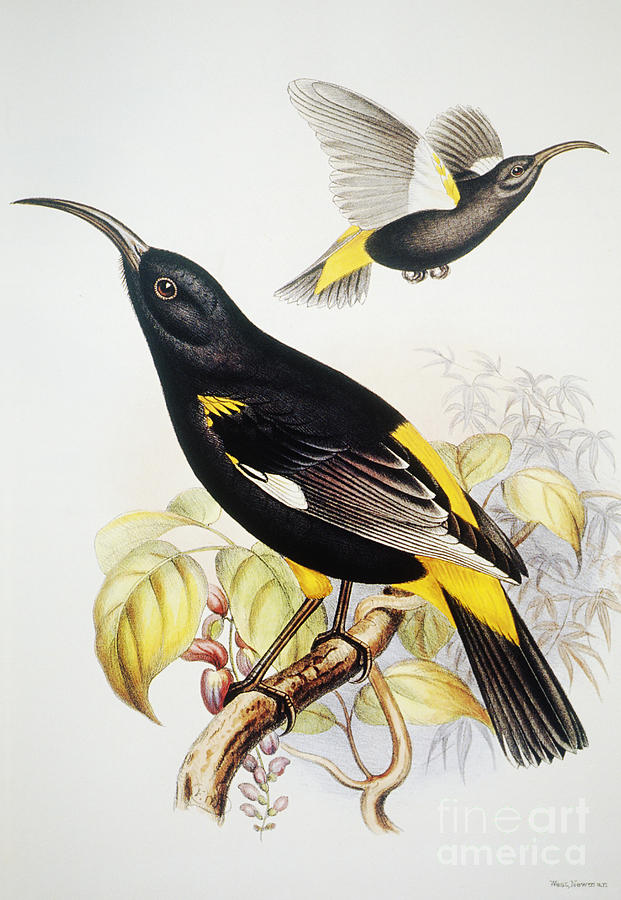This detailed painting features two black birds, likely of the same species. One bird is perched on a branch toward the bottom left of the image, facing left, while the other is captured in mid-flight in the top right, heading to the right. The birds are characterized by their long, sharply curved beaks. The perched bird showcases brown eyes with black irises and striking yellow triangular feathers at the top of its wings, with a mix of white and black at the wingtips and a blue tail that transitions into black midway. The yellow on the birds extends from their wing roots down the back, not quite reaching the tail, and the underside of their panels, which continues down to the middle of their tail feathers. Both birds also have gray wings, with some white near the roots. The branch, adorned with green leaves and small red petals, adds a contrasting background to the predominantly dark birds. The image also includes a watermark at the bottom reading "Fine Art America," and an artist’s signature that appears to read "West Newman" or "Newman West."